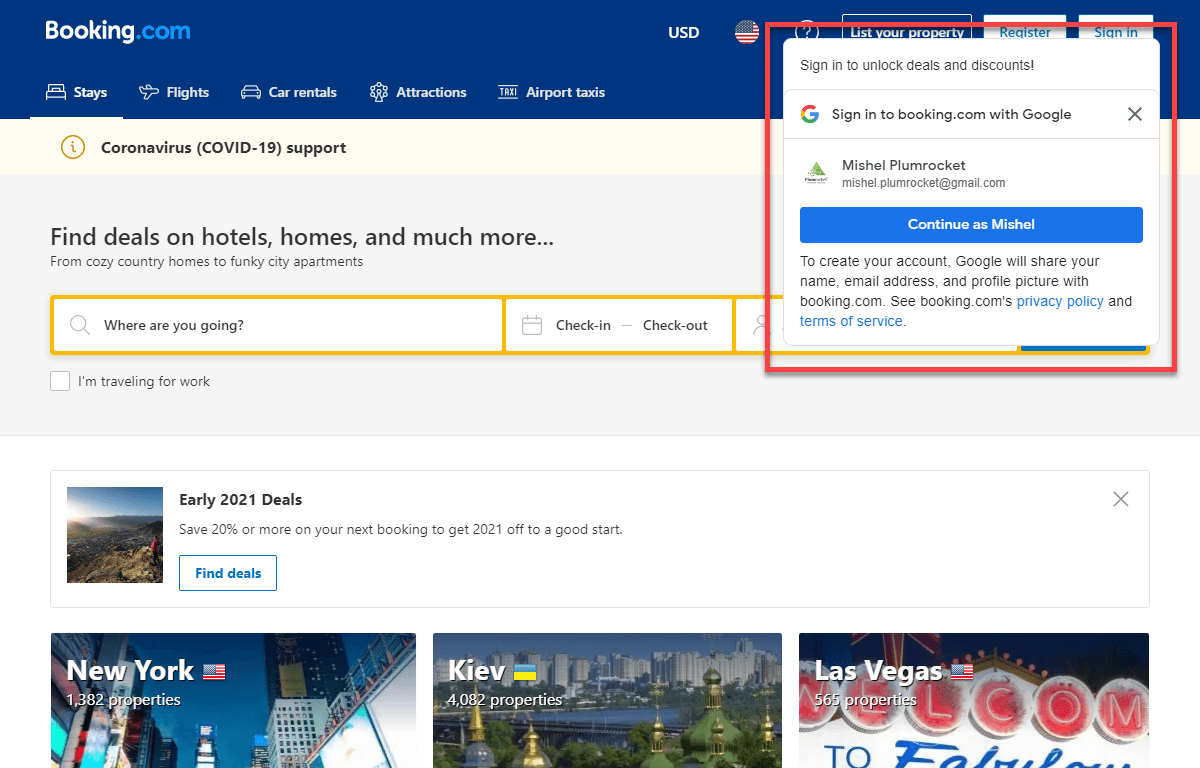The image depicts the homepage of the website Booking.com. On the right-hand side, a red-highlighted box draws attention to a sign-in prompt, displaying the message: "Sign in to unlock deals and discounts. Sign in to Booking.com with Google." Below this, the text includes a pre-filled name and email address: "Mishal Plumashay" and "mishal.plumashay@gmail.com", along with a button labeled "Continue as Mishal". There is an informational note that states, "To create your account, Google will share your name, email address, and picture with Booking.com. See Booking.com's Privacy Policy and Terms of Service for more details."  

In the background, the page header displays the text "USA, USD, USA", positioned towards the top-right. Centered towards the top are navigation options reading "Stays," "Flights," "Car Rentals," "Attractions," and what appears to be "Airport Tools." Just below this, a banner reads, "Coronavirus (COVID-19) Support," offering assistance related to the ongoing pandemic. Additionally, the site provides search options for entering a destination, along with check-in and check-out dates, which enable users to browse and book hotels, car rentals, flights, and various attractions. Booking.com appears to offer a comprehensive platform for securing a wide range of travel-related reservations, potentially featuring competitive deals.